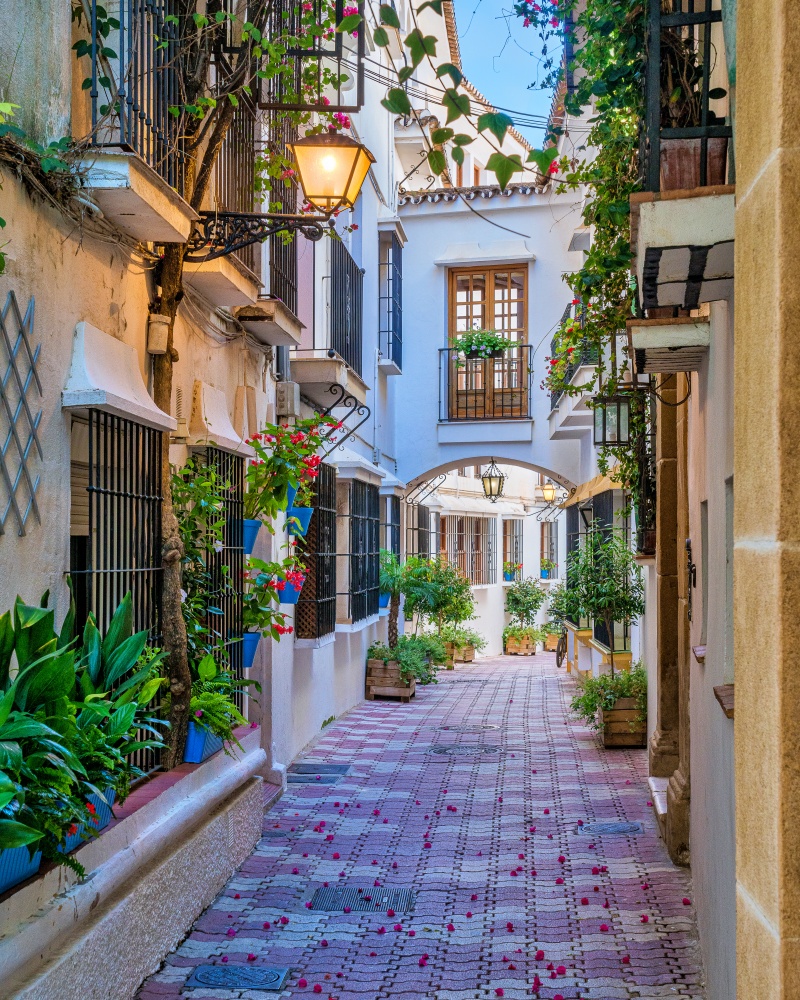The image depicts a vibrant, brightly colored alleyway reminiscent of Venetian architecture, featuring rows of closely positioned buildings facing each other. The paved walkway is composed of interlocked stones in hues of mauve, pink, and blue, interspersed with small metal grates. Scattered across the walkway are numerous small red and pink petals, possibly from nearby flowers. Lining the alley are decorative wooden boxes filled with a variety of plants, including shrubs, flowers, and hanging vines that add a touch of lush greenery to the scene. The windows of the houses are outfitted with wrought iron bars, painted black, adding a sense of security and style. One light, positioned in the upper left corner of the image, glows despite the daylight. An archway featuring a wooden balcony with potted plants adds architectural interest to the picturesque walkway. The absence of people and the presence of blue planters, power lines, and a clear blue sky above enhance the quaint and serene atmosphere of this charming alleyway.